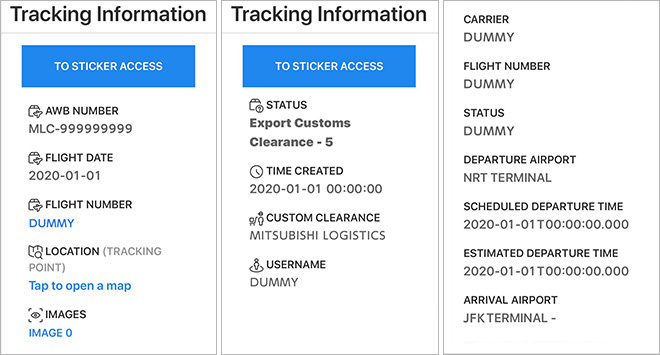The image features three distinct smartphone screens displayed from left to right against a white background, each showcasing detailed tracking information for a shipment. The most notable aspects include the consistent use of bold black lettering and a streamlined interface lacking any usual top bars.

The first screen presents the initial tracking details with a prominent blue clickable button labeled "Two Sticker Access." Below it, the AWB number is displayed, followed by the flight date of January 1st, 2020. The flight number is rendered in blue with the placeholder name "dummy." The location field indicates an option to open a map, but there are no images provided for the shipment.

On the second screen, the header remains "Tracking Information," with continuity in the button for "Two Sticker Access," maintaining the focus on shipment status. The status is marked as "Export Customs Clearance" with a timestamp of January 1st, 2020. Detailed entries such as "Customs Clearance" and "Mitsubishi Logistics" appear, while the username "dummy" is now displayed in grey. The term "Carrier" and all following information remain placeholders, emphasizing their dummy nature.

The third screen delves deeper into the shipment specifics. The carrier, flight number, status, and other pertinent details are all placeholders bearing the word "dummy." It lists the departure airport as NRT terminal with a scheduled departure date of January 1st, 2020, but without any specified time. Similarly, the estimated departure date is the same, not providing a precise time. The arrival airport is noted as JFK terminal, indicating the shipment's trajectory from Mitsubishi to New York, although it is still in the early stages of its shipping process.